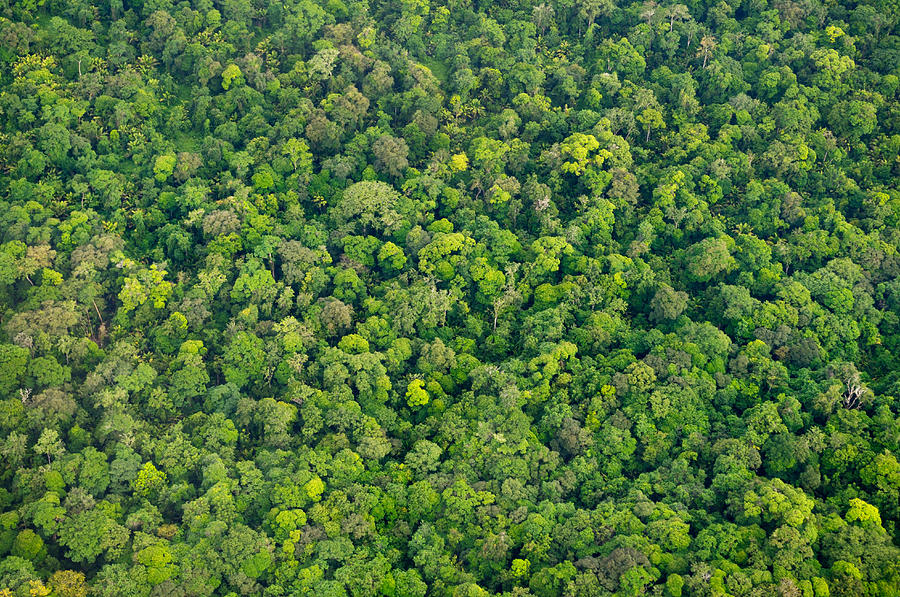This aerial naturescape photograph captures a dense forest filled with an endless expanse of trees in various stages of growth. The diverse shades of green—ranging from dark, rich greens to lighter, subdued tones—suggest different ages and types of trees, with some possibly younger and others older. Interspersed among the predominant greens are hints of yellow and brownish-green hues. The absence of walkable paths gives the impression of an untouched wilderness, hinting at the potential for getting lost if one were to venture into its depths. The image, taken during what appears to be springtime given the lack of evergreens, offers a fascinating view of the forest canopy. In the middle of the image, a small section reveals more of the tree branches, and a few tall, skinny trunks are visible. Small patches where trees are sparse allow glimpses of the ground below, resembling an up-close view of broccoli. The entire frame is devoid of any text, allowing the complex beauty of nature to command full attention.